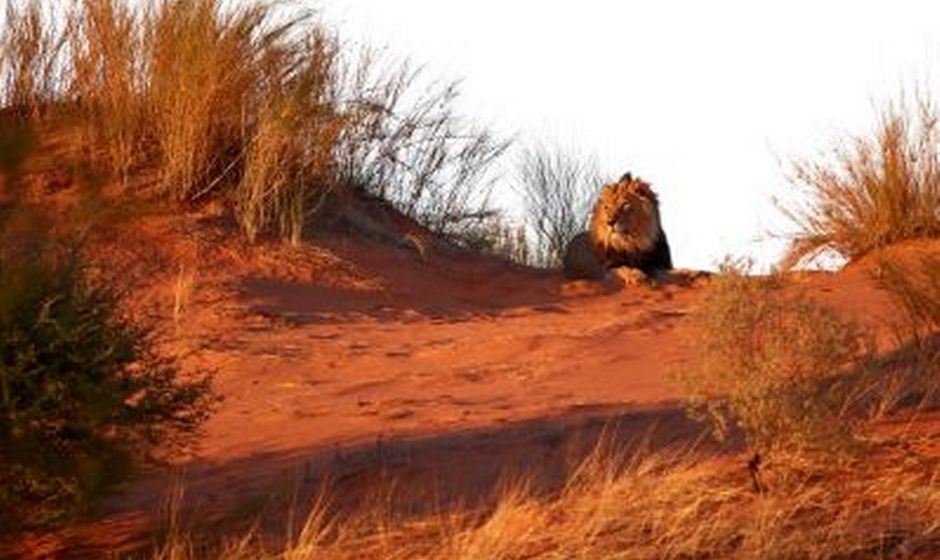In this landscape-oriented image, we see a majestic male lion lying atop a red, sandy hill, with his regal head held high. His massive mane, rich in dark and light brown hues, frames his face as he gazes contemplatively to the left. The lion's body reclines in the bright, orangish-red dirt, almost resembling a dirt road due to the cleared path around him. The scene is illuminated by the sun, casting long shadows and suggesting the time is either sunrise or sunset. Surrounding the lion, the landscape is dotted with dry grasses and brownish-green tall brush, adding to the arid atmosphere. In the bottom left, a green shrub stands out amidst the otherwise dry environment. The sky above is a nearly uniform white, covered by clouds, highlighting the starkness of the landscape. Overall, the picture evokes a tranquil yet striking scene, likely captured in the African wilderness.